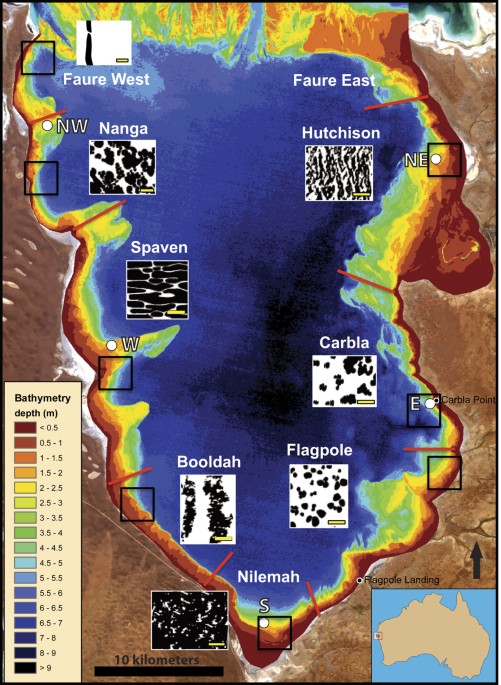This image illustrates a detailed topographical map titled "F-A-U-R-E West" and "F-A-U-R-E East" at the top left and right respectively. The map features several square highlights marking locations such as Nanga, Hutchinson, Spaven, Karbla, Bulda, Flagpole, and Neoma. At the bottom, Flagpole Landing is labeled in small black letters with a dot for its exact location. A key on the left explains the bathymetry depths, ranging from less than 0.5 meters in red to greater than 9 meters in black, passing through the colors of the rainbow. The map's depth colors transition through blue, green, yellow, and red. A scale indicating 10 kilometers is also present. An inset at the bottom right portrays a tan outline of Australia against a light blue background, suggesting the map's geographical context within Australian waters.